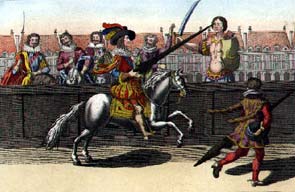The image depicts a lively, detailed scene from the Renaissance era, showcasing a jousting event. Central to the composition is a man on a white horse adorned with a fancy saddle and a gold blanket. The rider, dressed in deep red and gold medieval garments, wears an elaborate hat with three feathers—red, blue, and yellow—and brandishes a long sword. To his right, a man on foot, dressed in a brown outfit with red sleeves and red tights, appears to be retrieving or engaging with a joust. Surrounding them are several men, also dressed in ornate attire with white collars, waving their swords and weapons in the air, intensifying the action. In the background, an extensive castle with grey walls and red roofs stretches across the image, adding to the grandeur of the scene. Notably, spectators, possibly fellow jousters, on horses watch the duel, and one man stands out holding a green shield and a sword, witnessing the spectacle. The whole scene pulls from influences resembling the famous depiction of Antoine de Plevinals, rich with mustachioed and goateed men, further grounding the image in its historical setting.